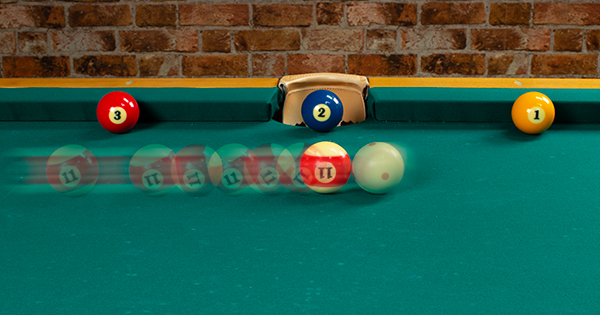This rectangular indoor photograph captures a dynamic moment mid-play on a green felt pool table, framed by a rustic brick wall in red and brown hues with gray grout. Central to the composition is a striking multi-frame motion effect, showcasing the white cue ball with red dots hitting the red-striped 11 ball, creating a ghostly, semi-transparent trail of the 11 ball's movement towards the left side of the image. The table is scattered with solid balls: the red 3 ball on the left, the blue 2 ball positioned just in front of the side pocket, and the yellow 1 ball on the right. The detailed scene is further accentuated by the wooden trim of the pool table and faint white chalk marks, adding to the sense of action and depth in this almost time-lapsed photograph.